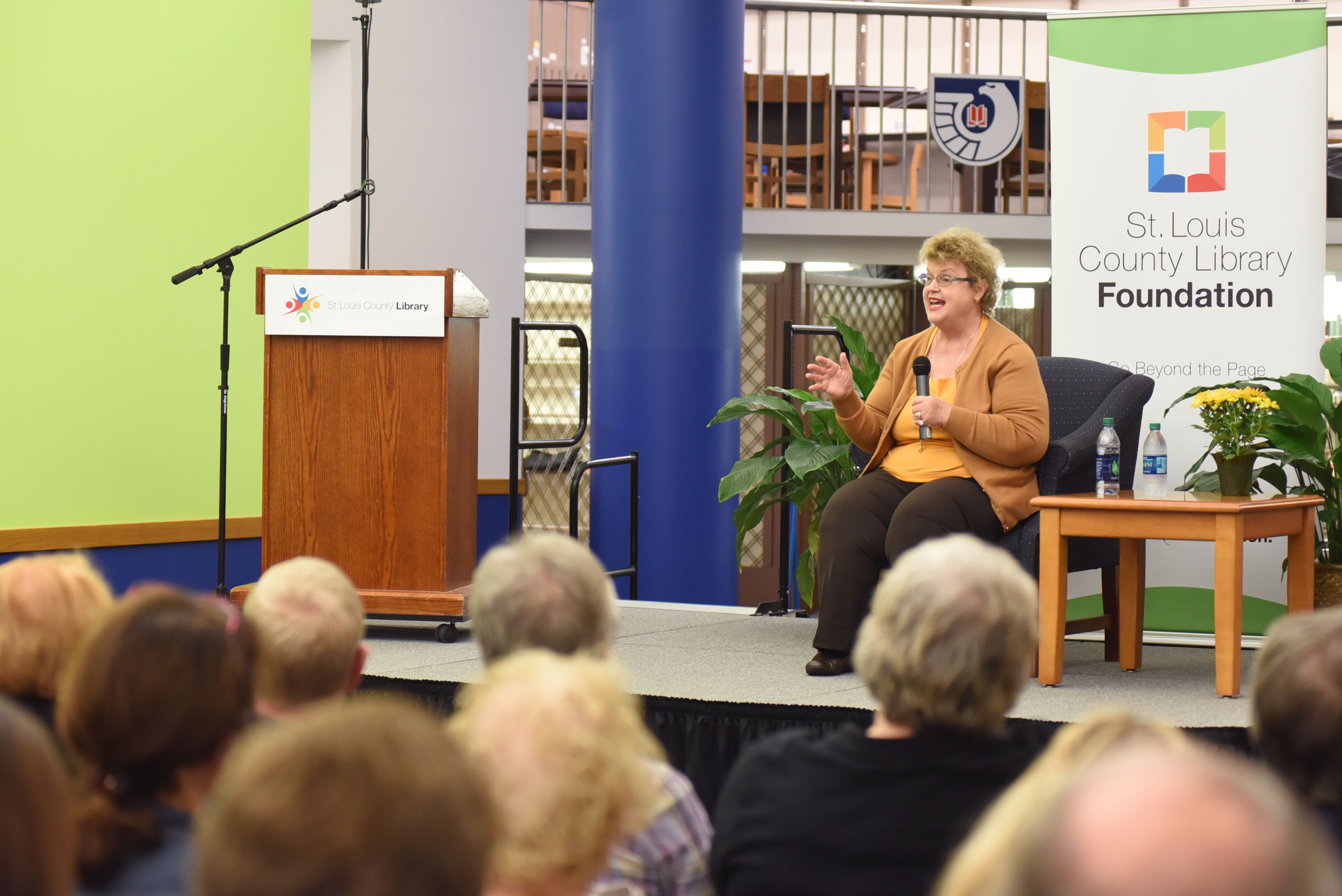The image captures a moment during a speech or presentation at the St. Louis County Library Foundation, held in what appears to be a library or similar public venue. Central to the scene is a middle-aged Caucasian woman, seated on a black chair on a stage, dressed in dark pants, a yellow-orange shirt, and a beige cardigan. She is holding a microphone in her left hand and gesturing expressively with her right. The woman has short curly hair and wears glasses. 

To her right, near the edge of the stage, stands a wooden podium with a white sign displaying the St. Louis County Library logo, which includes colorful emojis arranged in a circular pattern. A microphone is set up at this podium, although it is currently unoccupied. Behind the woman is a sign that reads "St. Louis County Library Foundation: Go Beyond the Page," featuring a square divided into four colorful quadrants—green, red, blue, and yellow. 

Next to the speaker, there is a small table adorned with bottles of water and a pot of flowers. In the background, a blue column can be seen, and above the stage area, railings and additional tables and chairs suggest the presence of a second tier or balcony. The audience, consisting of middle-aged or older individuals, attentively listens to the speaker, though the photograph reveals only a portion of the crowd, indicating that more than nine people are in attendance.